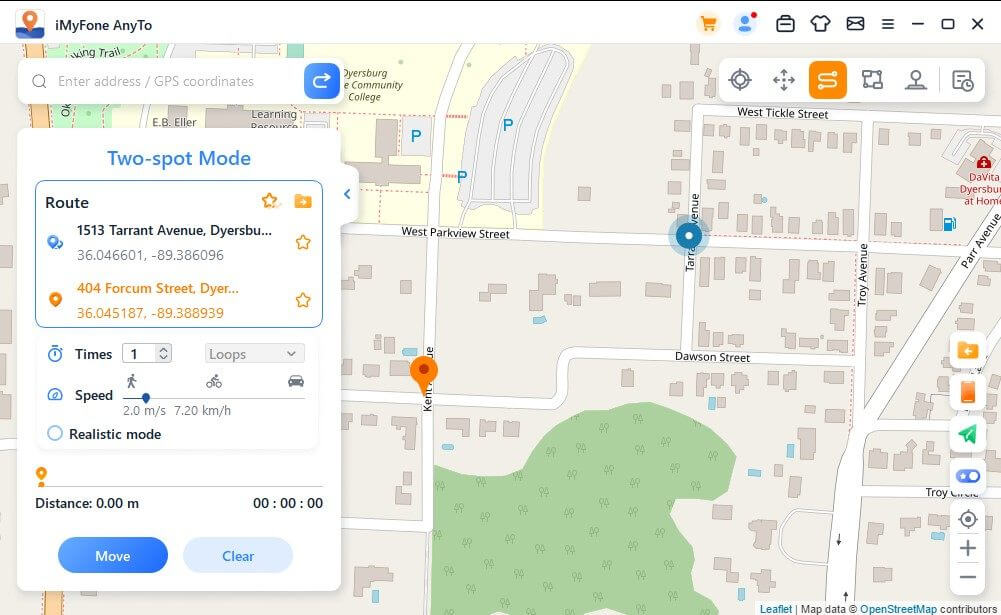This image is a screenshot depicting the user interface of a mobile app designed for phone location tracking. In the upper left-hand corner, there is a pen icon commonly associated with navigation and mapping software. The app's name is displayed prominently at the top of the screen as "iMyFONE AnyTo.”

Beneath the pen icon, there is a search bar labeled "Enter address or GPS coordinates," allowing users to input specific locations. The central part of the screen features a detailed map that highlights a pinned destination, along with an additional location marker. This map includes visible details such as streets, buildings, and green areas, providing a clear visual context of the surroundings.

On the left side of the screen, there is a modal menu titled "Two-Spot Mode," allowing users to perform various functions such as calculating the route, determining time, measuring speed, and assessing the distance between locations for precise navigation and planning.